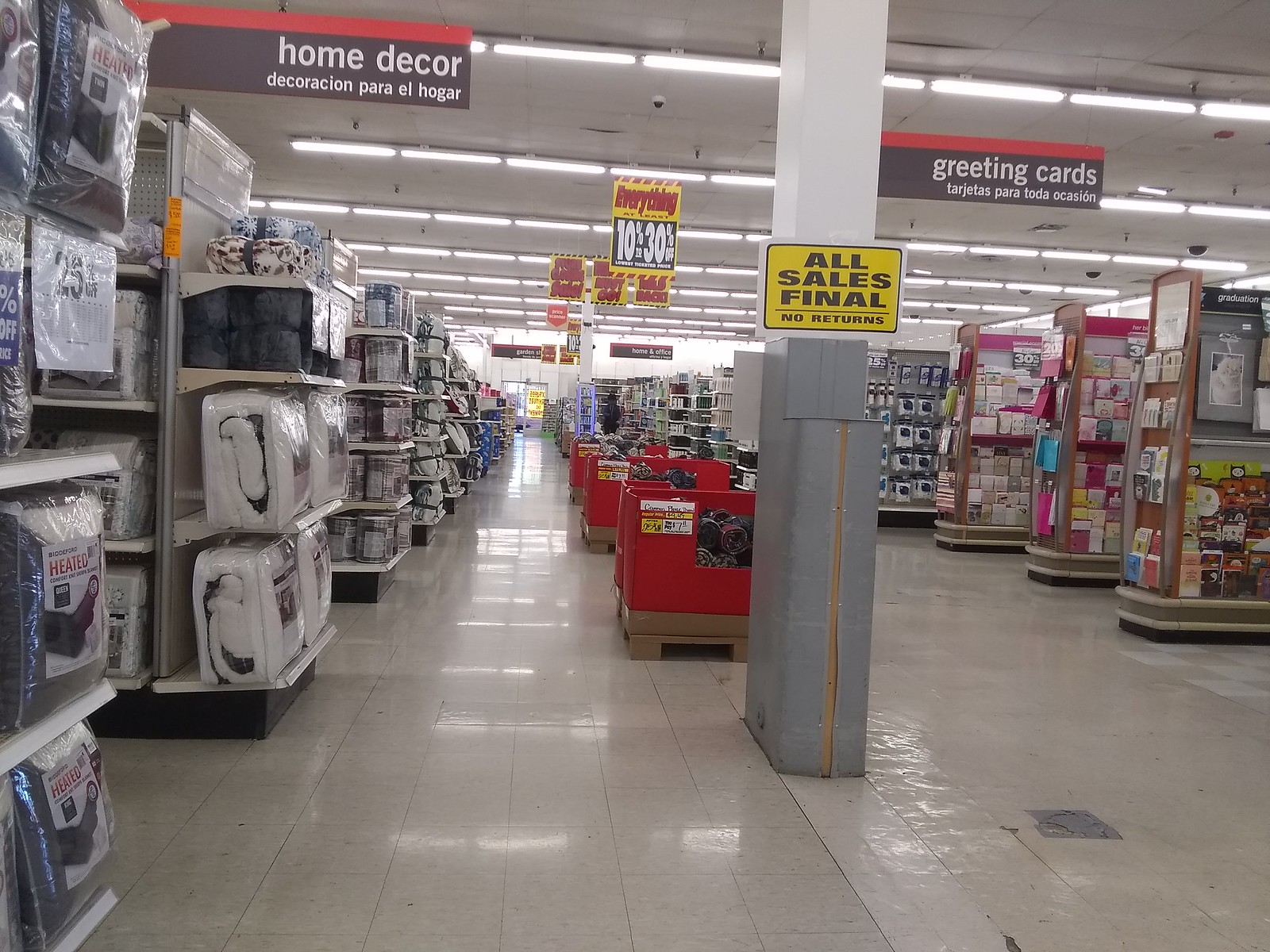The image depicts the interior of an unidentified store. Dominating the foreground is a metal post with a prominent yellow sign that has white edging and reads "ALL SALES FINAL NO RETURNS" in bold, black, all-capital letters. Further composed towards the back, another sign partially visible, appears to read "EVERY DAY, EVERYTHING..." although the specifics remain unclear. Adjacent to the original post, there’s an additional sign reading "Greeting Cards" alongside text in another language, likely Spanish. Similarly, on the upper left-hand side, a sign indicates "Home Decor," also accompanied by text in another foreign language. Below this sign, there are rows of shelving stocked with various bedding items. The floor throughout the store is covered in beige tiles. Center to the image, several bins can be seen, presumably filled with miscellaneous goods. Background elements include additional signage and more shelving units stocked with various items, although the exact nature of these items remains indistinguishable. Overall, the store is characterized by organized but closely packed aisles and various categories of merchandise.